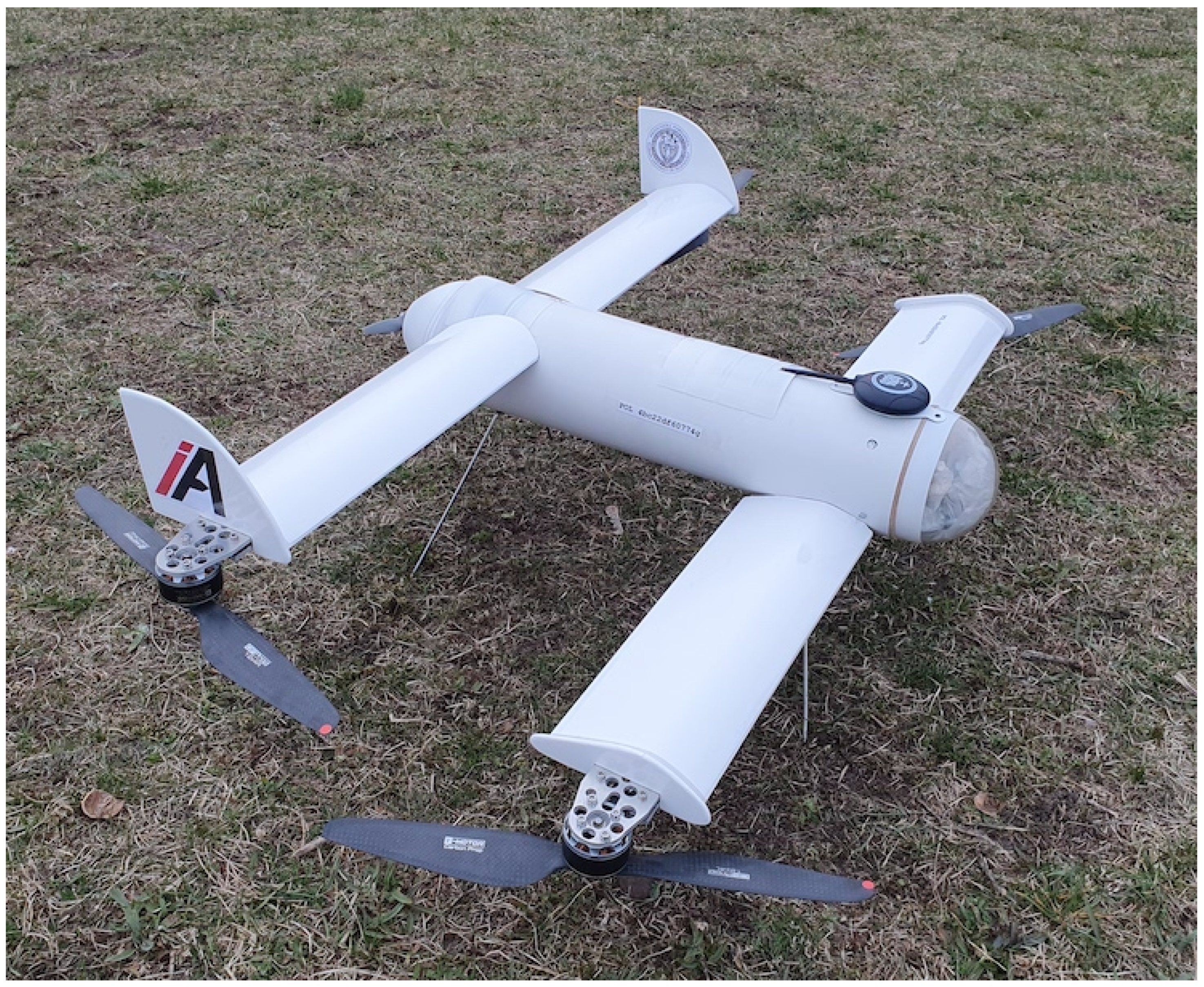The image depicts a small white drone, crafted from hard plastic with some metallic components. The drone features a central cylindrical body with four wings extending horizontally—two at the front and two at the back. Each wing is equipped with black rotors and silver-and-black motors, likely made from stainless steel, designed to propel the device. The front portion of the drone is adorned with a clear glass dome, while the top exhibits a black disc with an antenna protruding from it. Notably, the left wing bears a distinct logo composed of a red lowercase 'i' and a black uppercase 'A'. The drone is positioned on a patchy, dry grassy surface, where yellow, brown, and occasional green patches of grass are visible.